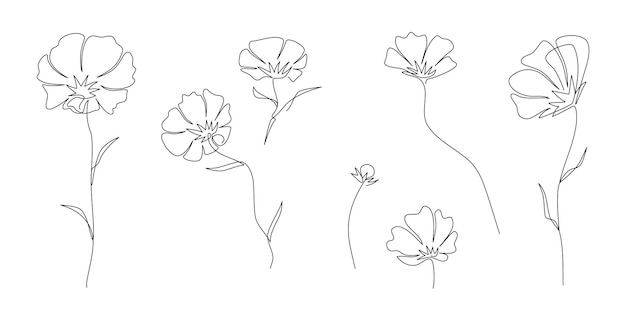The image features a finely hand-drawn arrangement of flowers, each rendered in a grayish pencil or charcoal on a solid white background. The drawing includes seven flowers in total, each with distinct characteristics. The first flower on the left has two leaves on its stem, multiple petals, and a star-like center. Next to it, another flower also has two leaves and has petals that bend slightly to the left. Above and shorter than these, a third flower also has two leaves but is drawn higher up. Diagonally to its right, there is a very small bloom with no leaves. Below and to the right of this tiny flower, a larger bloom emerges with barely any visible stem but with discernable petals. To the right of this, a long-stemmed flower without leaves and with four petals stands out. Finally, the furthest to the right features a flower with two withered petals, leaves on the stem, and facing leftward. These floral sketches, featuring simple lines and arranged in varying heights and positions, create a strikingly minimalist yet detailed botanical study on a stark white backdrop.